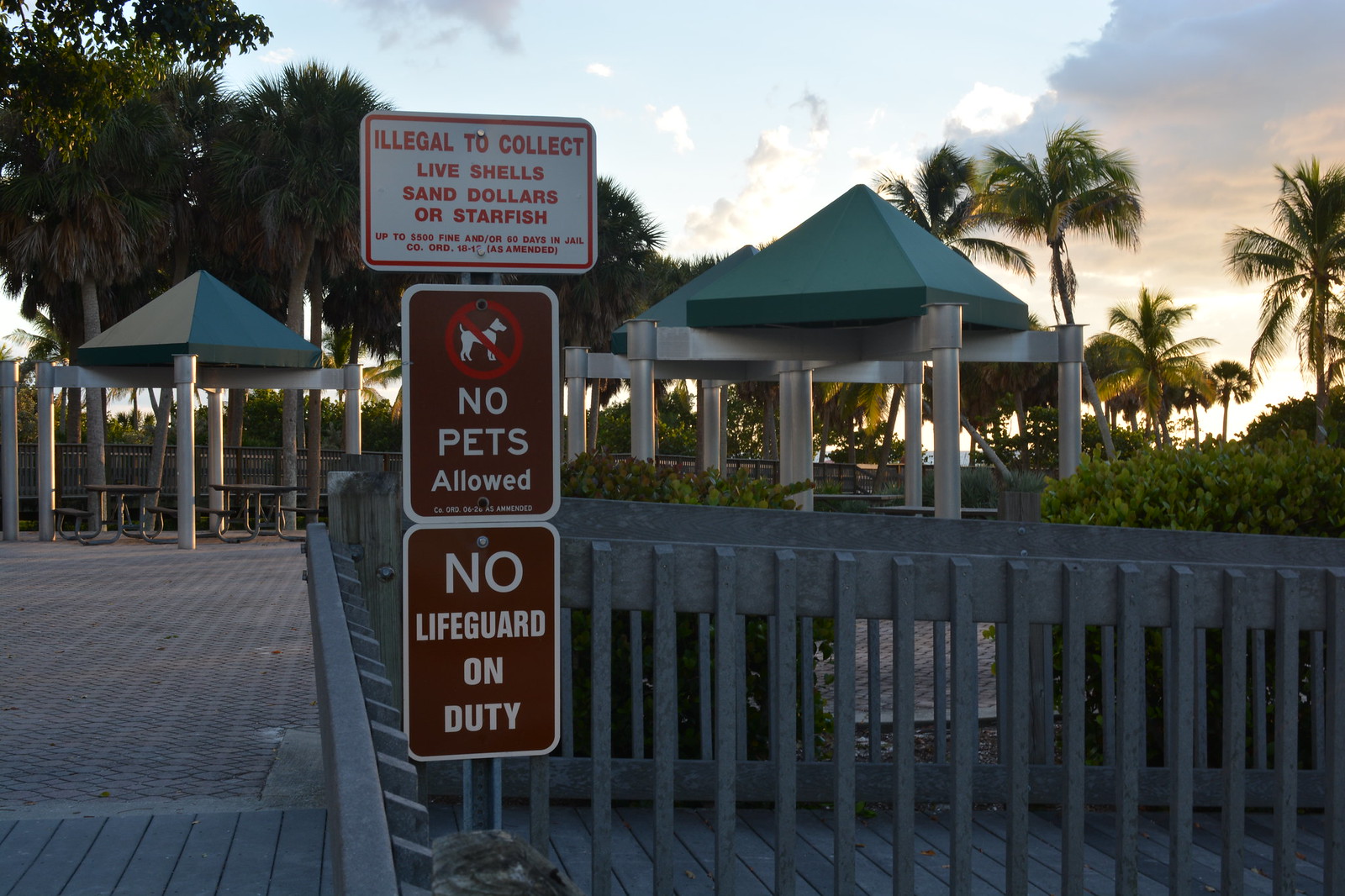The image depicts an outdoor beach entrance area at sunset, featuring a wooden boardwalk with light gray railings. Prominently displayed at the entrance is a sign with three notices: the top white sign stating it's illegal to collect live seashells, sand dollars, or starfish, with a penalty of up to $500 fine or 60 days in jail; a middle brown sign indicating "No Pets Allowed" with a dog crossed out; and a bottom brown sign warning "No Lifeguard on Duty." Beyond the sign, there's a paved area with several green, pyramid-shaped metal awnings over picnic tables and benches. The scene is surrounded by beach bushes and palm trees, contributing to the coastal atmosphere.